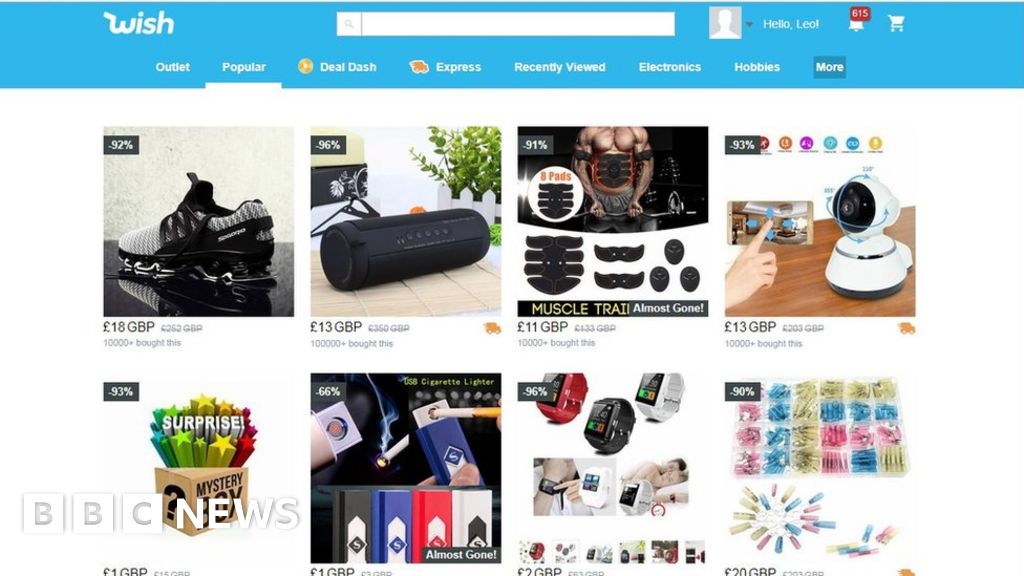This is a detailed description of a cropped screenshot depicting the Wish website's homepage. The image captures the top portion of the page, prominently featuring a blue header. On the top left, the recognizable Wish logo is displayed centrally. To the right of the logo, a search bar is located, followed by a blank user profile photo. Adjacent to the profile photo, it greets the signed-in user with a "Hello Leo" message. 

On the far right of the header, there is a bell icon accompanied by a red notification badge showing the number 615, indicating the user has 615 alerts. An icon of a shopping cart is positioned to the right of the notification bell.

Immediately below the header, a navigation bar showcases various categories listed horizontally along the bottom of the blue header bar, including "Outlet," "Popular," "Deal Dash," "Express," "Recently Viewed," "Electronics," "Hobbies," and "More." The "Popular" category is currently selected, highlighted by a white underline.

The main body of the webpage features a clean white background displaying eight product thumbnails in a grid format. Each product listing includes its price at the bottom along with the number of purchases made underneath the price.

In the bottom left corner of the screenshot, there is a white watermark of the BBC News logo, indicating the source of the image.